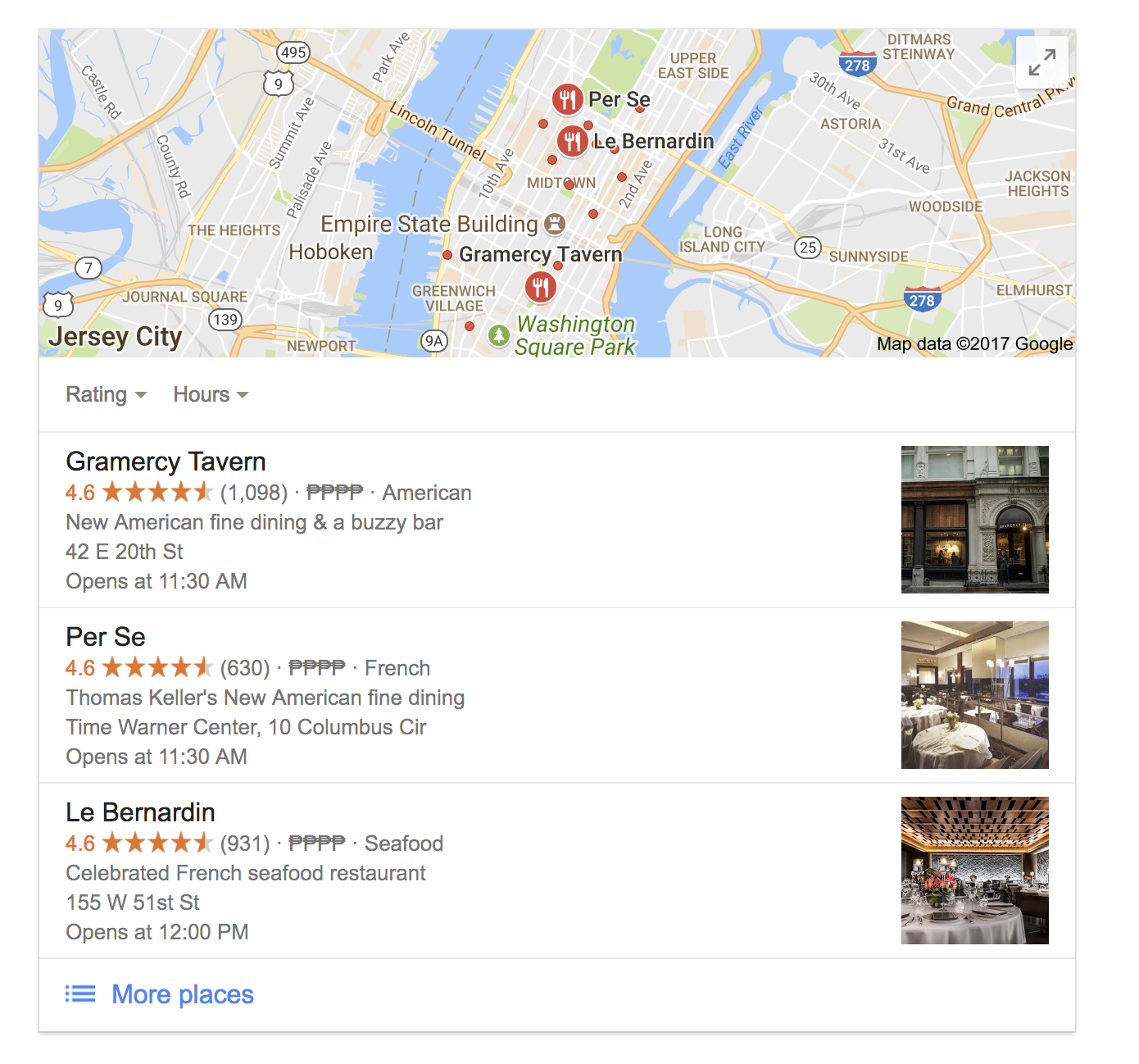This is a screenshot of a Google search for dining locations that prominently features a map at the top. The map, which fills the entire upper section, displays multiple red pins with fork and knife icons, indicating different dining establishments.

Below the map, there is a white background section that begins with filters for ratings and hours on the top left, each accompanied by a drop-down menu for sorting the search results.

The main content features a vertical list of dining businesses matching the pins on the map. The first listing is for "Gramercy Tavern." The detailed format for each entry includes the restaurant's name at the top, followed by its star rating and the number of reviews in parentheses to the right. Adjacent to this, there is a gray flag icon with four flags displayed. Further to the right, the type of cuisine is specified as "American."

Beneath these details, there is a short description of the restaurant, its address, and the opening time, listed as "opens at 11:30 AM." A square thumbnail image of Gramercy Tavern is positioned on the right side of the listing.

This format is consistently followed for all the businesses in the search results, with each entry having a thumbnail on the right and descriptive details on the left. At the bottom left corner of the screenshot, the text "more places" in blue suggests additional listings are available but not visible in this cropped view, which includes only the map and the first three restaurant listings.